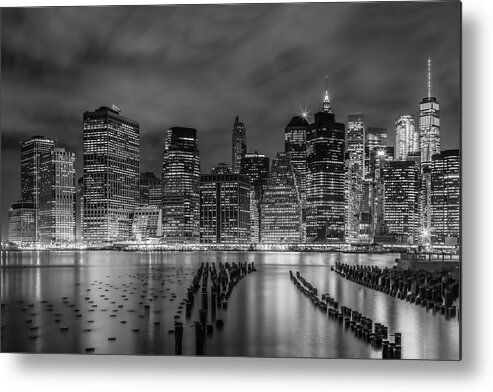This black-and-white photograph captures a mesmerizing city skyline at night. The image, which is rectangular in shape and framed, features a vast collection of illuminated skyscrapers standing tall against a backdrop of a cloudy, gray night sky. In the lower third of the photo lies a tranquil body of water that reflects the city's lights, adding a serene quality to the scene. Dotting the water are evenly spaced protruding wooden posts, creating a rhythmic pattern from the left to the right side of the frame. The entire composition, from the shimmering buildings to the still water and scattered posts, exudes a captivating contrast between architectural brightness and the calm darkness of the night.